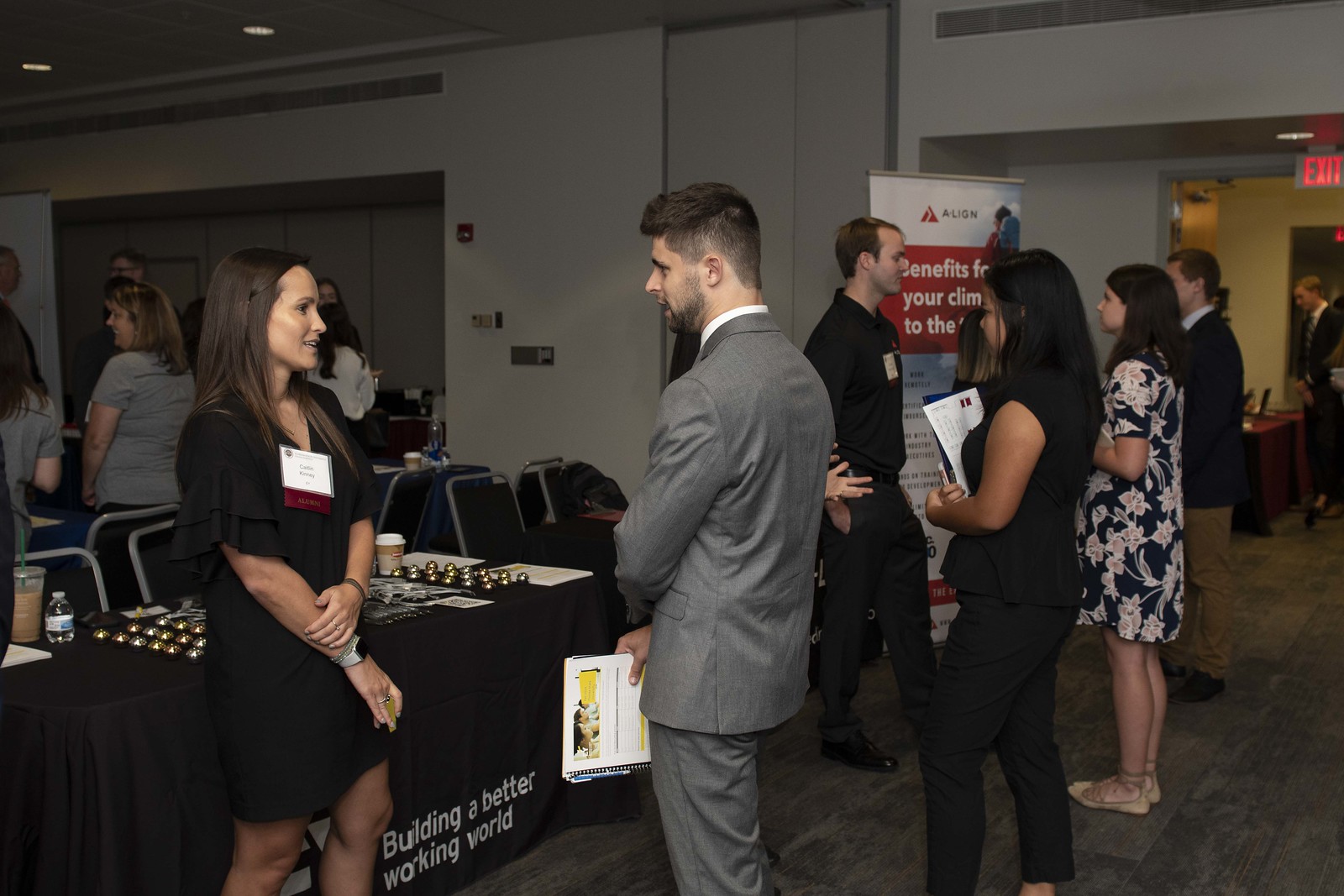In a bustling hotel conference room, attendees can be seen engaging in lively discussions. Central to the scene is a large rectangular table draped in a black cloth emblazoned with the words "Building a Better Working World." The table is laden with various items, including a plastic water bottle, a beverage in a plastic cup, a covered to-go coffee cup, and several papers. 

Standing in front of this table, a woman dressed in a black dress with a name tag pinned to her front engages in conversation with a man in a gray suit, who has a beard and holds some papers. Both are positioned about three feet apart, with their arms crossed in front of them, maintaining eye contact. The woman is accessorized with a watch on her right wrist and bracelets on her left. 

In the background, there's a pedestal with banners and multiple groups of people, including two women and another mixed-gender pair involved in their discussions. The area exudes the collaborative spirit of a trade show, further emphasized by a sign that reads, "Benefit Your Climb to the Top."